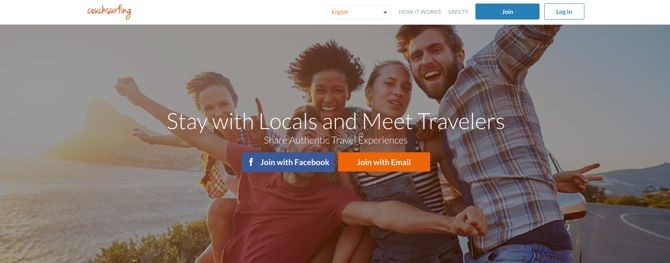The image is a screenshot from a holiday accommodation website, likely Couchsurfing, given the name displayed in a small, cursive red font at the top left corner. The majority of the screenshot showcases a vibrant, full-page background photograph of a lively group of five young people at a beachside holiday destination. The group, which includes a bearded man, a young white woman, a black girl, another man, and another girl, all share a moment of joy with their arms around each other, smiling and cheering with their arms raised.

Prominently placed across the middle of the image is a welcoming message: "Stay with locals and meet travelers," with a subheading, "Share authentic travel experiences," just below. Below this invitation are two interactive boxes for joining the site: a blue box labeled "Join with Facebook" featuring the Facebook icon, and an orange box labeled "Join with Email."

At the top of the page, several navigation options are visible. A language selection drop-down is highlighted in red with English as the default language. Next to it, black tabs read "How it works" and "Safety." To the right, there are two more boxes for account actions: a blue "Join" box with white text and a "Login" box with blue text on a white background framed by a blue border. This visually engaging website is designed for travelers looking to connect and share genuine travel experiences with locals.